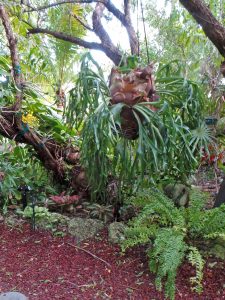This image depicts a lush and meticulously maintained tropical or summertime backyard garden brimming with vibrant greenery. The scene is populated with various trees bearing wide, multi-parted leaves and long, stringy fronds. The sunlight filters through the dense foliage, creating a dappled effect on the reddish, mulch-covered soil below. Amongst the greenery, yellow flowers bloom on a tree branch to the left, while red flowers add a pop of color to the right-hand side.

The foreground features a delineated path of wood chips bordered by stones, suggesting both intentional landscaping and a clear walkway. Succulents are planted near the ground, adding to the garden's diverse plant life. Your attention is drawn to an intriguing element hanging from a tree, which appears to be a brown object ensconced in rope, lush with surrounding green leaves—resembling either a plant in a tree pot or some form of decorative garden ornament.

Overall, the image captures a bright, sunny day with glimpses of a grayish-blue sky through the abundant tree canopy, showcasing a beautifully maintained garden that blends natural abundance with cultivated order.